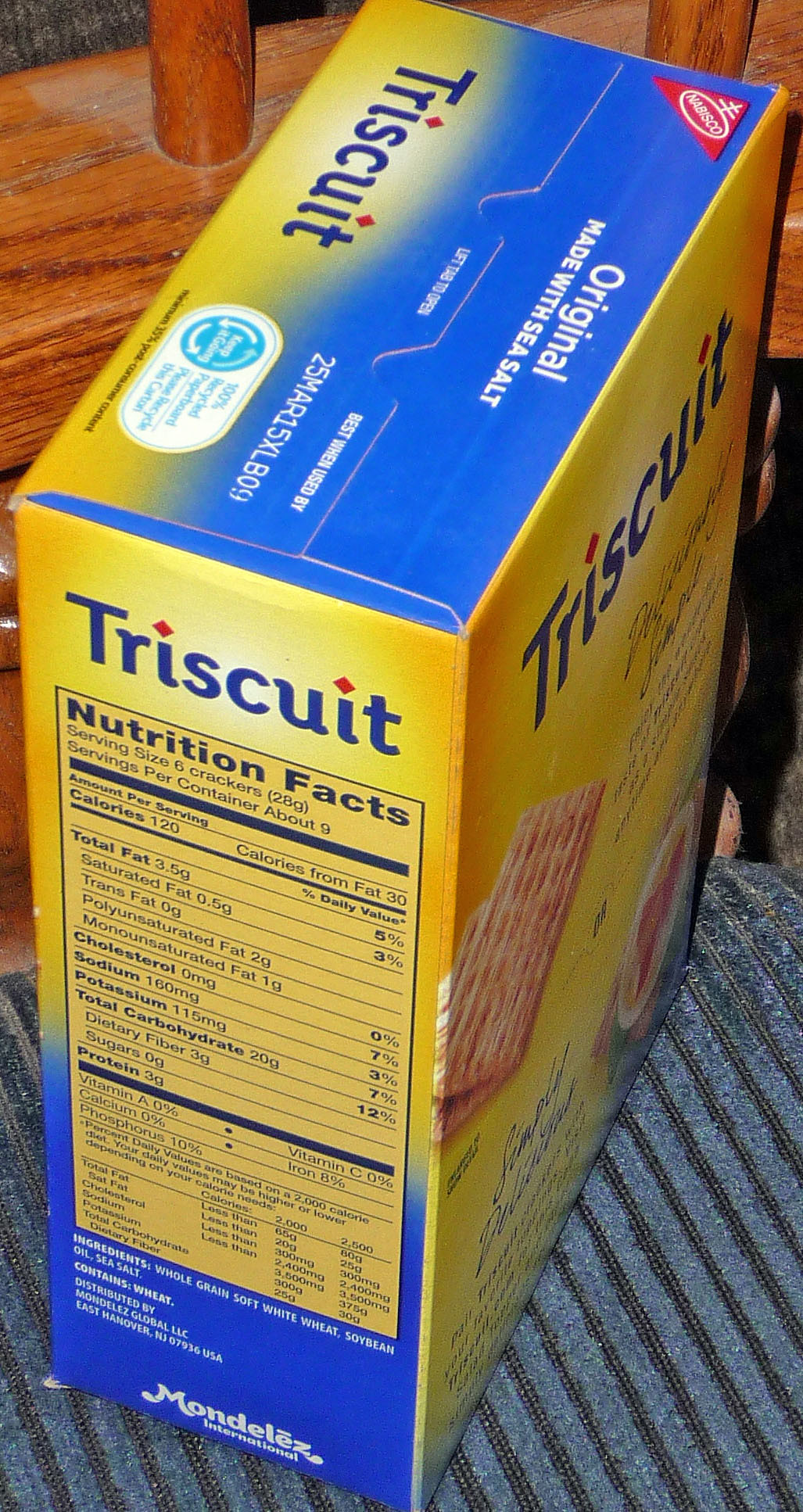This vertical image showcases a sealed box of Triscuit crackers. The box is primarily yellow with blue accents and is positioned at an angle, displaying the top, the nutrition facts on the side panel, and part of the back. The top of the box, which says "Original Made with Sea Salt" and displays the Nabisco logo, is oriented upside down due to the angle. The nutrition facts are prominently shown on the side panel in a tabular format on a yellow background with black text, indicating that the serving size is 20 grams (about 6 crackers), totaling 120 calories per serving.

The word "Triscuit" appears multiple times, including on the top and back panels, with a distinctive diamond-shaped red accent above the 'i'. The back panel also displays photographs of the crackers against the yellow background. The box is situated on a blue upholstered chair with darker, bluer, and grayer lines for division, against a background of finished wood with some dust, possibly showing a table or a cabinet in the back.